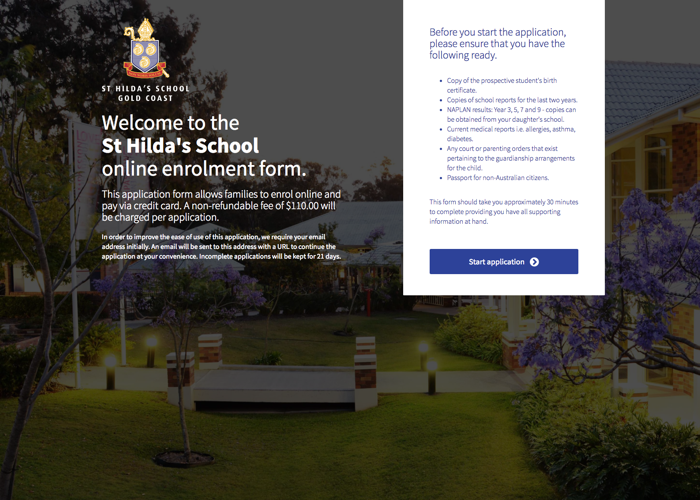A screenshot displays the tranquil grounds of a college campus, captured in the gentle evening light. Brightly lit pathways meander among lush trees, some adorned with purple flowers while others showcase vivid green leaves. Nestled amidst the verdant scenery, a building stands alongside a tent bearing the banner "St. Hilda's School Gold Coast." The banner welcomes visitors to the St. Hilda’s School Online Enrollment Form, detailing the steps for families to enroll online and process payments via credit card, including a non-refundable fee of $110 per application.

On the right side of the image, a white rectangular box outlines essential preparatory steps for applicants. The instructions, highlighted in blue, advise families to have several documents ready: a copy of the prospective student's birth certificate, school reports from the past two years, NAPLAN results for years 3, 5, 7, and 9 obtainable from the daughter’s school, and current medical reports for conditions such as allergies, asthma, or diabetes. The serene environment and meticulous instructions aim to facilitate a smooth enrollment process for prospective students.